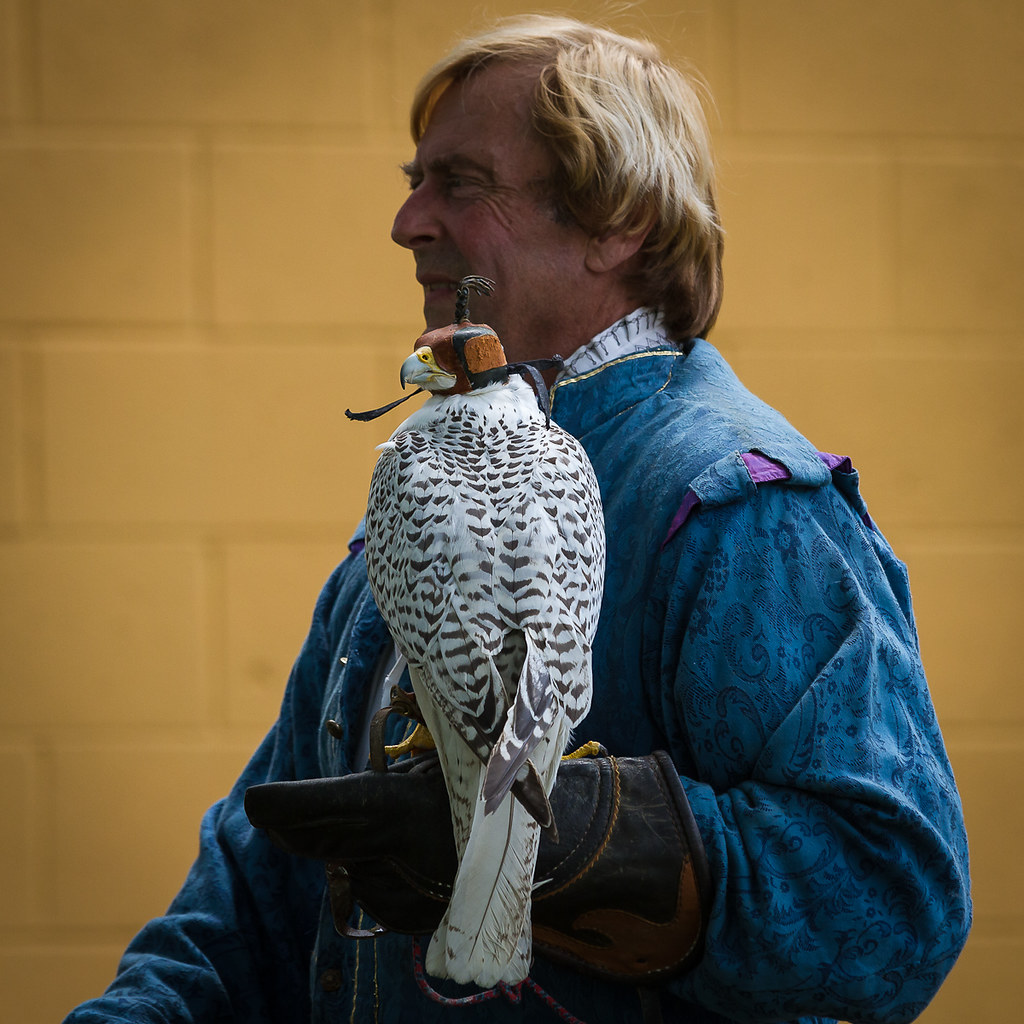The image is a professional-quality photograph of a man holding a bird, likely a falcon or a kite. The man, who has medium-length brownish-blonde hair, a pointy nose, and a smiling face marked with wrinkles, is dressed in an ornate blue tunic-style outfit with billowy long sleeves and a patterned surface. He is standing against a yellow brick wall. On his left hand, which is protected by a heavy black leather glove, perches the bird. The bird, white with grey and black markings, has its back partially turned to the camera and wears a hood or cap covering its eyes, indicative of its training. The detailed depiction of both the man and the bird highlights the intricate dynamic between a falconer and his avian companion.